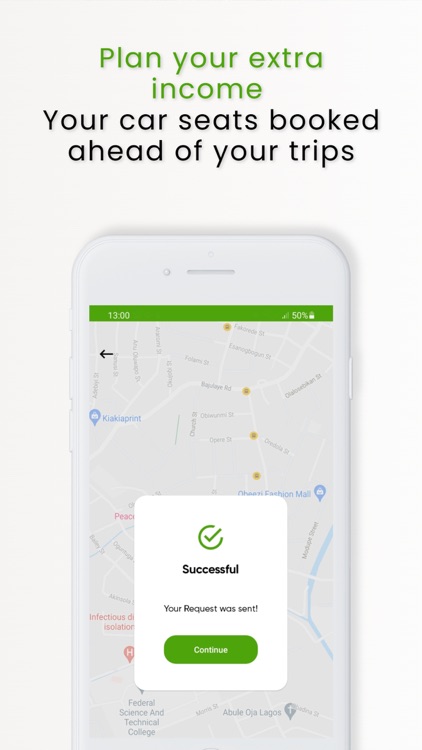The advertisement prominently features the slogan "Plan Your Extra Income, Your Car Seats Booked Ahead of Your Trips" at the top. Below this text, a sleek white iPhone is displayed, indicating a time of 13:00 with the battery at 50%. The phone screen showcases a map background, with an overlay of a white pop-up box in the center. The pop-up, emphasized by a vivid green check mark, reads "Successful your request was sent" and includes a green "Continue" button. The map's details are blurred out, focusing attention on the pop-up message. The slogan suggests a dual function: not only can users plan to earn extra income, but they can also ensure their car seat arrangements are managed ahead of their trips. The clean and minimalistic design of the ad draws attention to the ease and efficiency of the service offered.